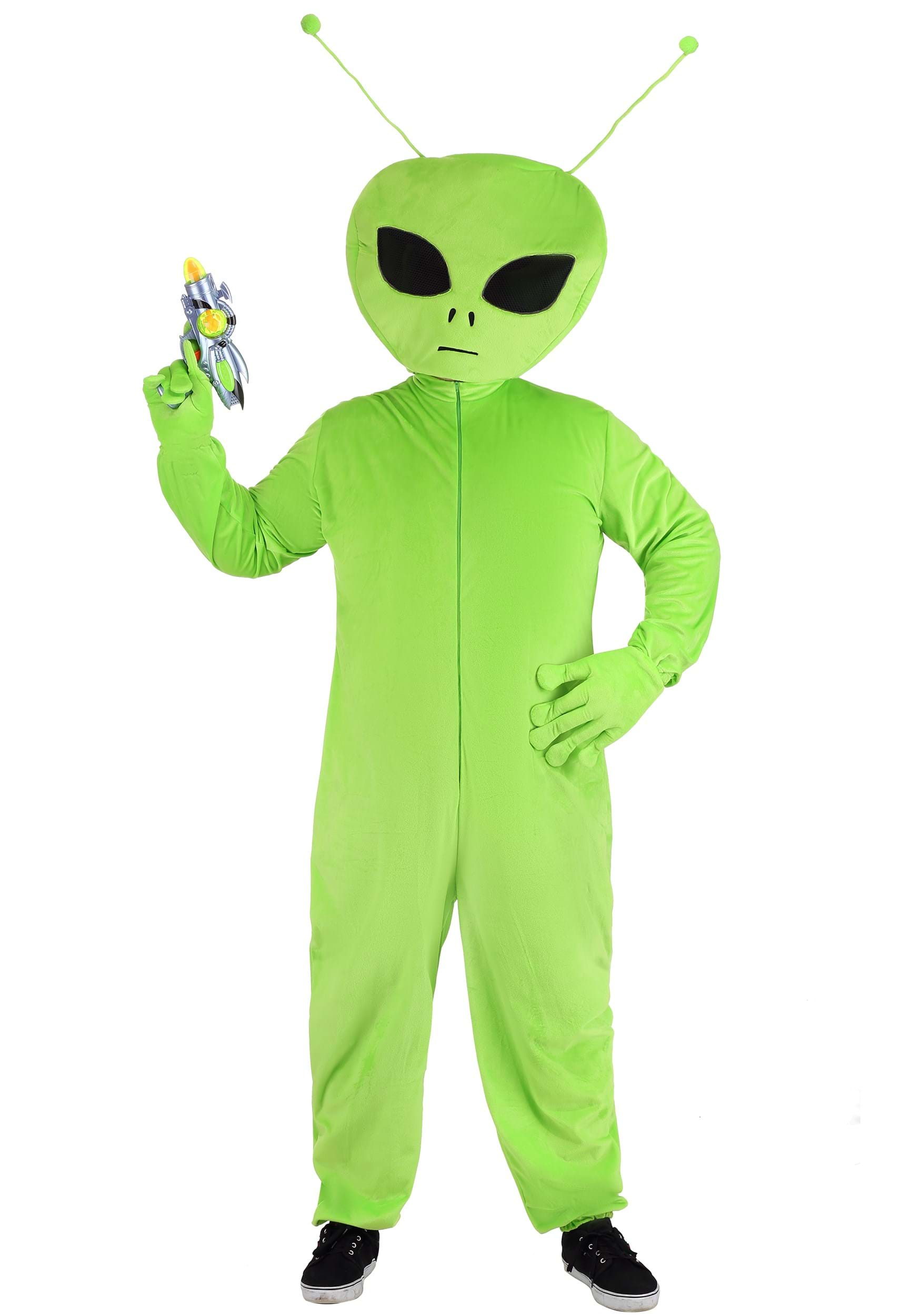The image depicts a child dressed as an alien in an advertisement-style setting with a pristine white background. The costume features a lime green tone, including a headpiece that forms a rounded, upside-down teardrop-shaped head with large black eyes, two small nostril slits, and a straight mouth slit. Protruding from the head are two thin green antennas with small balls on the ends. The outfit is likely made of velour or crushed velvet, encompassing a onesie that zips down the front and extends to both full-length sleeves and legs. Neon green gloves with bulbous fingertips match the suit, and black sneakers with white soles complete the ensemble. The child, striking a confident pose, has their left hand on their hip and their right hand holding a laser gun pointed upwards. This intricate design, from the matching green mask and gloves to the added accessory of the blaster, suggests the costume is intended for a Halloween or other themed event.